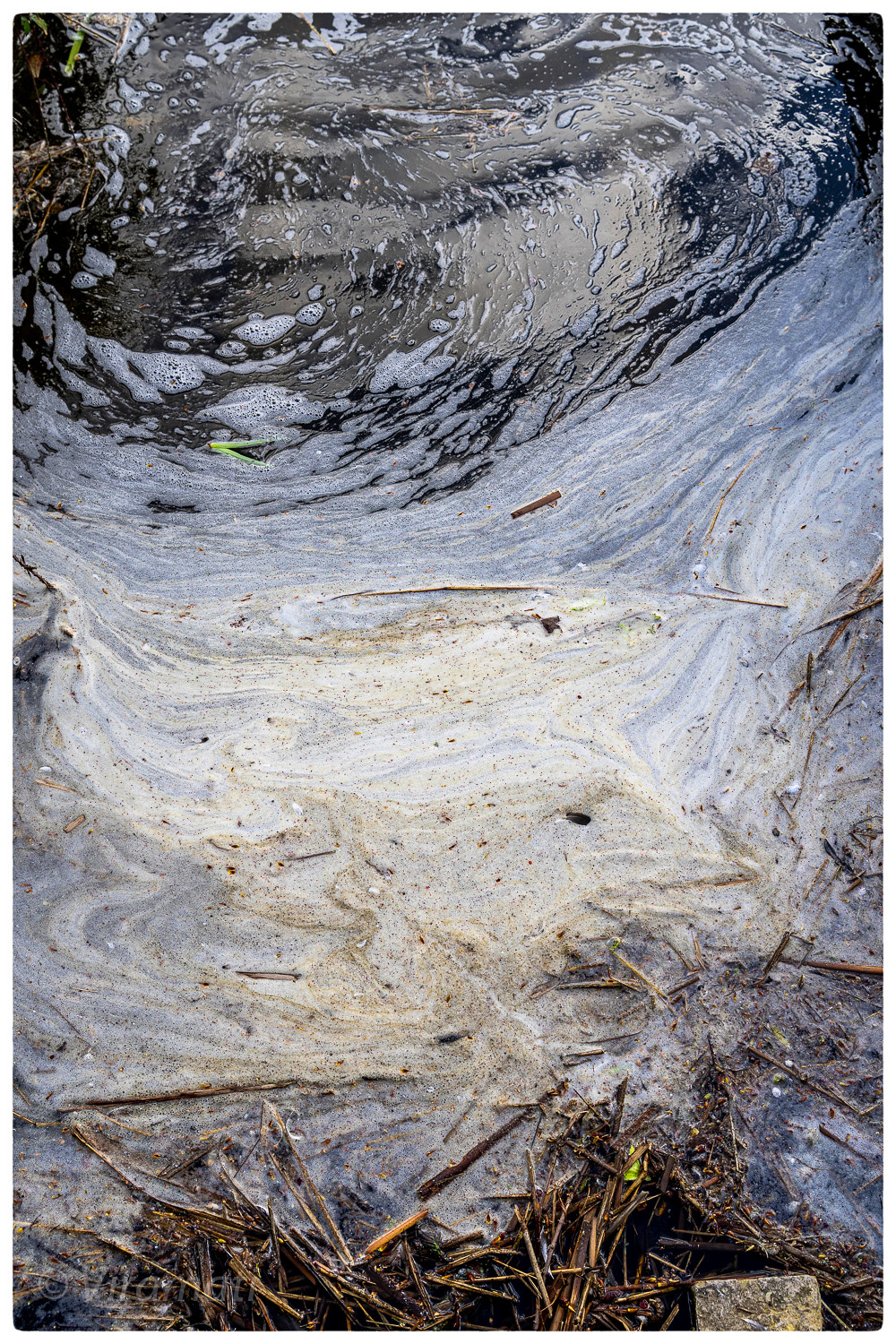The photograph captures an outdoor, daytime scene from a standing perspective, looking down at the edge of a polluted body of water. The rectangular image prominently features a swirl of off-colored, cream-colored foam floating on the water's surface, indicative of pollution. Along the shore, at the bottom of the image, straw or dead grass debris is piled up, likely washed up by the water. Among the debris, a piece of wood can be seen in the bottom-right corner. The photograph's colors include black, white, gray, green, yellow, and tan, with the water taking up most of the image. The water appears more clear as it extends away from the shore, although patches of foam persist. The scene conveys a sense of dirty, stagnant water, possibly resultant from chemical runoff or flooding, with an overall impression of an unappealing, hazardous environment.